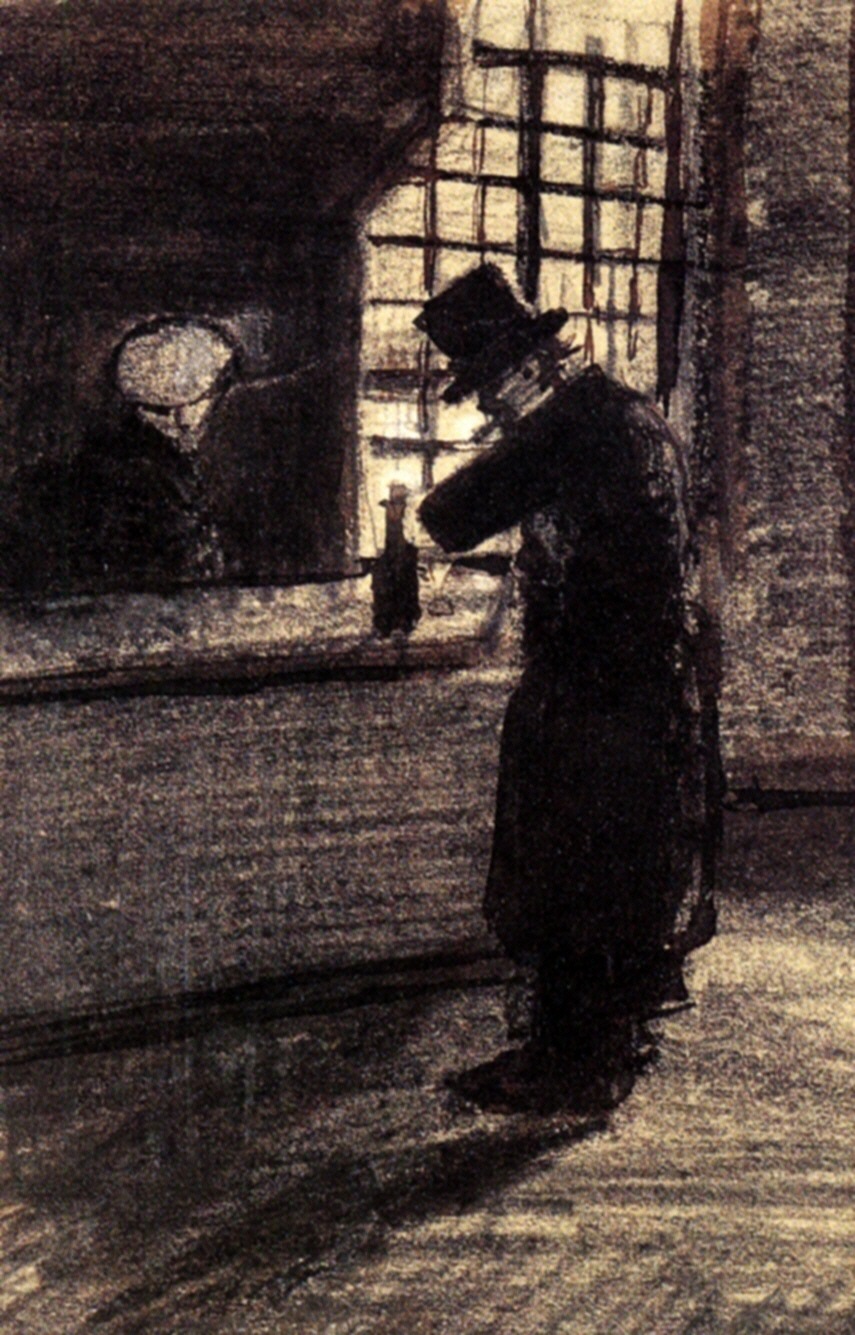This artwork, titled “Man in a Village Inn” from 1883, appears to be a charcoal or crayon print on a light to dark-toned paper, depicting a 19th-century scene inside an inn. Central to the image is a man in a black top hat and a knee-length, dark coat, his face obscured by the rough and impressionistic style of the medium. The man stands at the inn's bar or front counter, where a bottle—possibly of wine—rests.

To the left of the man, there’s a rectangular window through which soft light filters in, casting a shadow that gives depth to the scene. The window features visible support beams. The floor below the man is composed of broad swathes of dark color, enhancing the room's sparse and somber atmosphere. Behind the bar, a ghostly figure in a flat cap, its body indistinct, appears to gaze at the man, suggesting a transaction taking place. The man's left hand is busy with something at his mouth, possibly money or a cigar, while his right hand reaches into his coat pocket.

The scene is framed only by the two men, the bar, and perhaps a round object hanging on a wall, leaving the rest of the inn starkly empty, capturing a moment of isolated interaction rooted in its historical context.